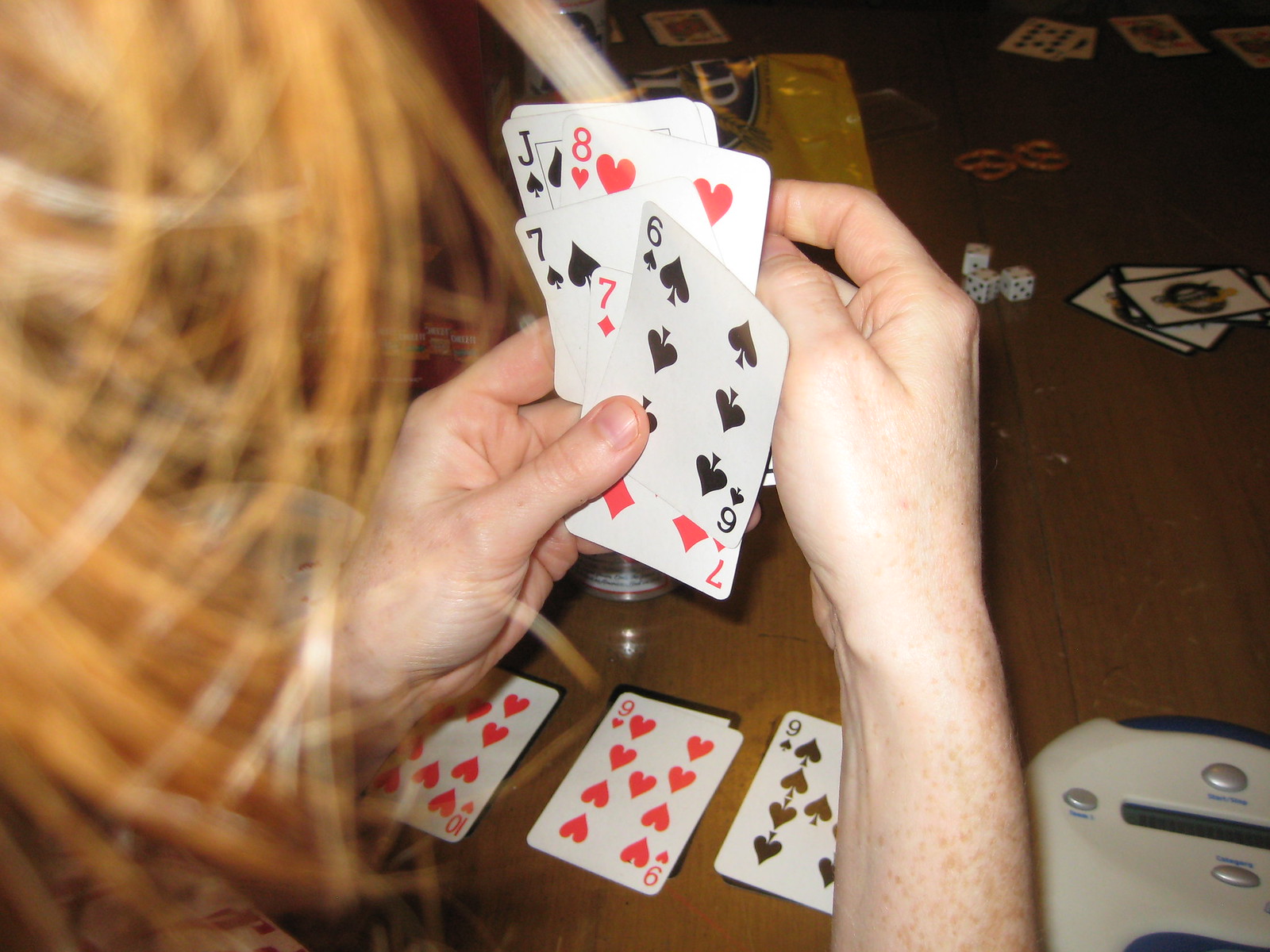A medium brown wooden table is the centerpiece of this image, adorned with various items indicative of a game night. Central to the arrangement is a yellow snack package, possibly a pretzel brand, featuring a black circle with white lettering. Scattered around the table are playing cards and dice, suggesting an ongoing card game.

Towards the right side of the image, a man with blurred long red hair is partially visible. His hands, Caucasian with freckles, hold a fan of cards: the six of clubs, seven of diamonds, seven of clubs, eight of hearts, and the jack of clubs. On the table before him lie the ten of hearts, nine of hearts, and nine of clubs.

Additionally, a white and blue electrical device with four silver buttons is positioned near the man, though its purpose remains unclear. In the shadowy background, more playing cards are visible, indicating the presence of other players around the table. The scene is a lively depiction of a leisurely card game at twilight.